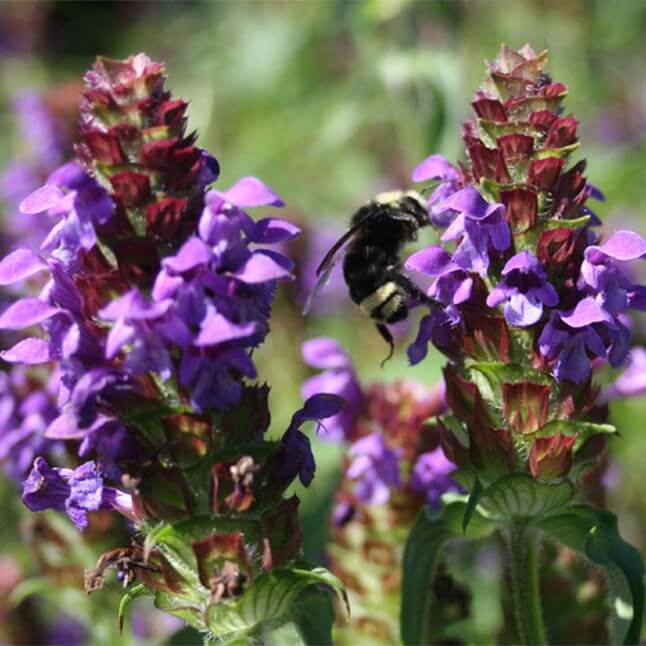In this vibrant, square-shaped color photograph taken in bright sunlight, two striking wildflowers stand prominently in the foreground. The flowers, possibly a type of salvia, have an orchid-like shape with vivid purple petals and some hints of dark red and green. Each flower emerges elegantly from a green stalk, reaching upwards. A bumblebee, characterized by its mostly black body and yellow head, is seen drinking nectar from the flower on the right, adding a dynamic touch to the scene. The background, although blurred, reveals a lush garden setting with more of these purple flowering plants and various greenery punctuated by occasional brown tones, enhancing the focus on the two main flowers and creating a vivid contrast. The overall composition captures the natural beauty and delicate details of the flowers and their environment, making it a stunning showcase of these wild plants in their natural habitat.